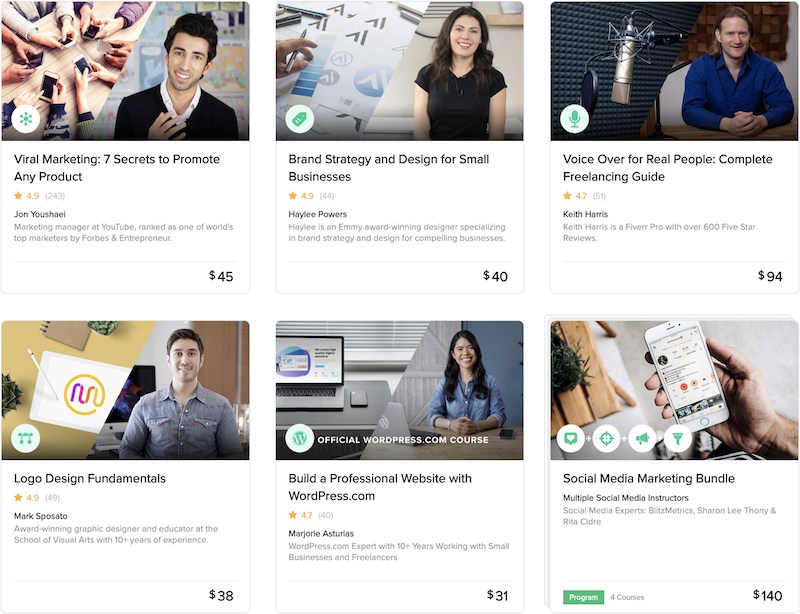The image displays six square article thumbnails, each showcasing a different online course. The first thumbnail highlights a course titled "Viral Marketing: Seven Secrets to Promote Any Product," which boasts 4.9 stars across 243 reviews and is priced at $45. The second thumbnail features an image of a woman and promotes a course on "Brand Strategy and Design for Small Businesses," also with 4.9 stars but from 44 reviews, and it's available for $40. The third course, "Voice Over for Real People: Complete Freelancing," has 4.7 stars from 51 reviews and costs $94. The fourth thumbnail is for "Logo Design Fundamentals," rated 4.9 stars from 49 reviews and priced at $38. The fifth course is titled "Build a Professional Website with WordPress.com," has a rating of 4.7 stars from 40 reviews, and costs $31. The final thumbnail advertises a "Social Media Marketing Bundle," priced at $140. A green rectangle on the image has the word "Program" written in white text, while in gray text it indicates that it includes four courses.